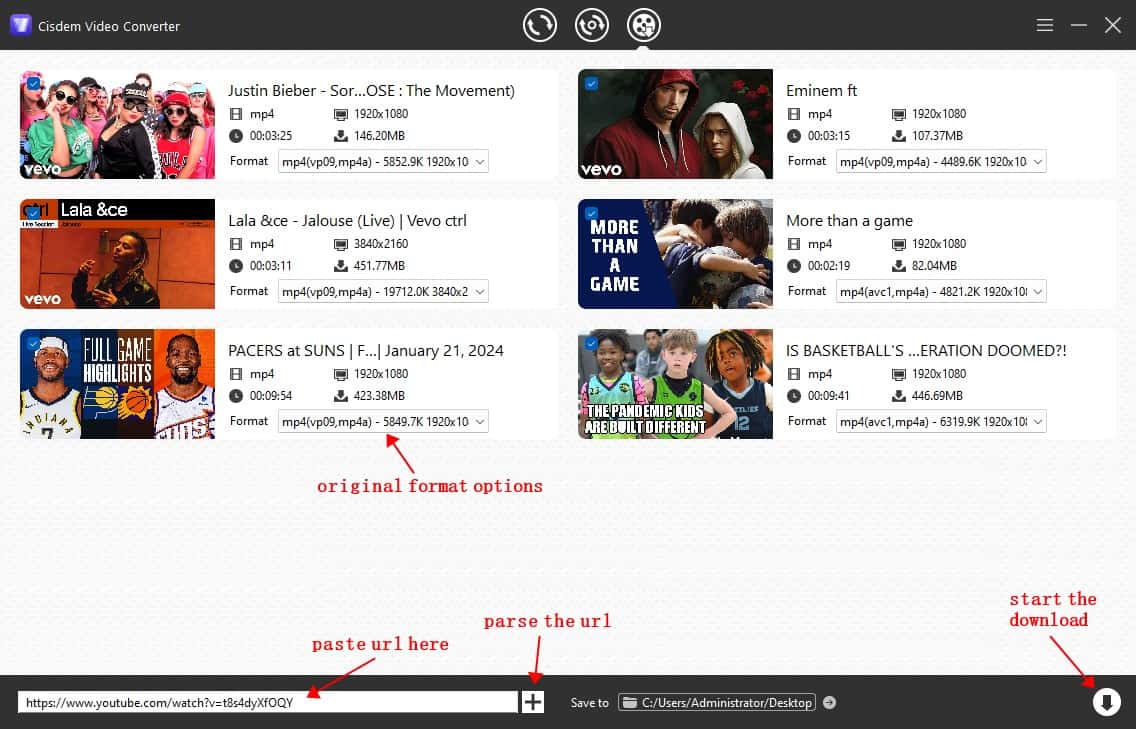This screenshot captures the interface of a website dedicated to video conversion and viewing. At the top, the header is highlighted with a black border featuring a prominent purple 'V' icon on the left, labeled "System Video Converter." Adjacent to this, three circular icons are lined up: the first shows two arrows forming a circular arrow, the second combines this circular arrow with a central dot, and the third displays a film reel icon. 

On the upper-right corner, there is a menu represented by three horizontal lines for additional options, alongside the standard window control buttons to minimize and close the application.

Below the header, the main interface showcases six video thumbnails, each accompanied by descriptions. The videos listed are:

1. Justin Bieber, "Sariose"
2. The Movement, "Eminem FT, Lala, and CE"
3. J-Lo, "Salao, Live Vivo Control"
4. "More Than a Game: Pacers and Sons"
5. "January 21st, 2024" 
6. "Is Basketball's Oration Doomed?"

Below the video listings, there's a section for selecting video formats labeled "Original Format Options," accompanied by a format dropdown menu. Additionally, input fields are provided to paste URLs, specifically from YouTube (e.g., youtube.com/watch URL), with a plus icon to parse the link.

Towards the bottom, there is an area labeled "Save To," indicating the destination, followed by a directory path labeled "Administrator.stopSaveTo." Finally, a prominent download button is situated in the bottom right-hand corner, allowing users to start the conversion and download process.